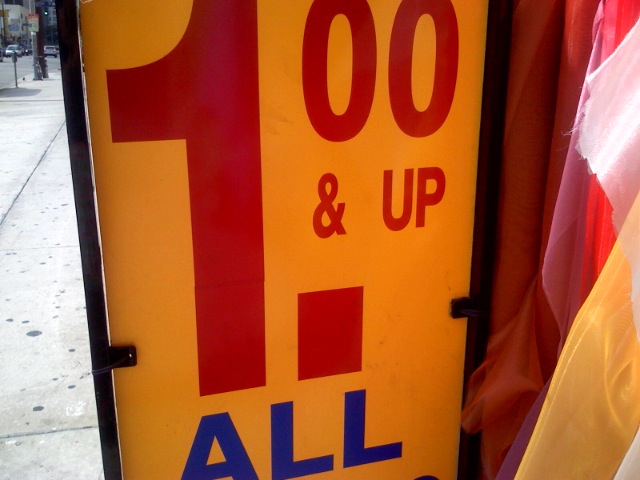The image features a zoomed-in view of a sign located outside, with portions of its text cut off due to the close-up perspective. The sign is framed in black metal on both the left and right sides and has an orange background. Prominently displayed in large red text is "$1 and up." The dollar sign and the numeral "1" are significantly larger than the surrounding text. Two zeros are positioned at the top of the sign, which seems off-centered. Below the "$1" is a red ampersand followed by the word "up." A small red square appears as a period beneath this text. Further down, in blue uppercase letters, is the word "ALL." Along the right edge of the image, various colorful pieces of cloth are visible, featuring gold, red, pink, and white colors. On the left side of the image, part of the sidewalk is seen, and in the distant background, there are cars moving in different directions.